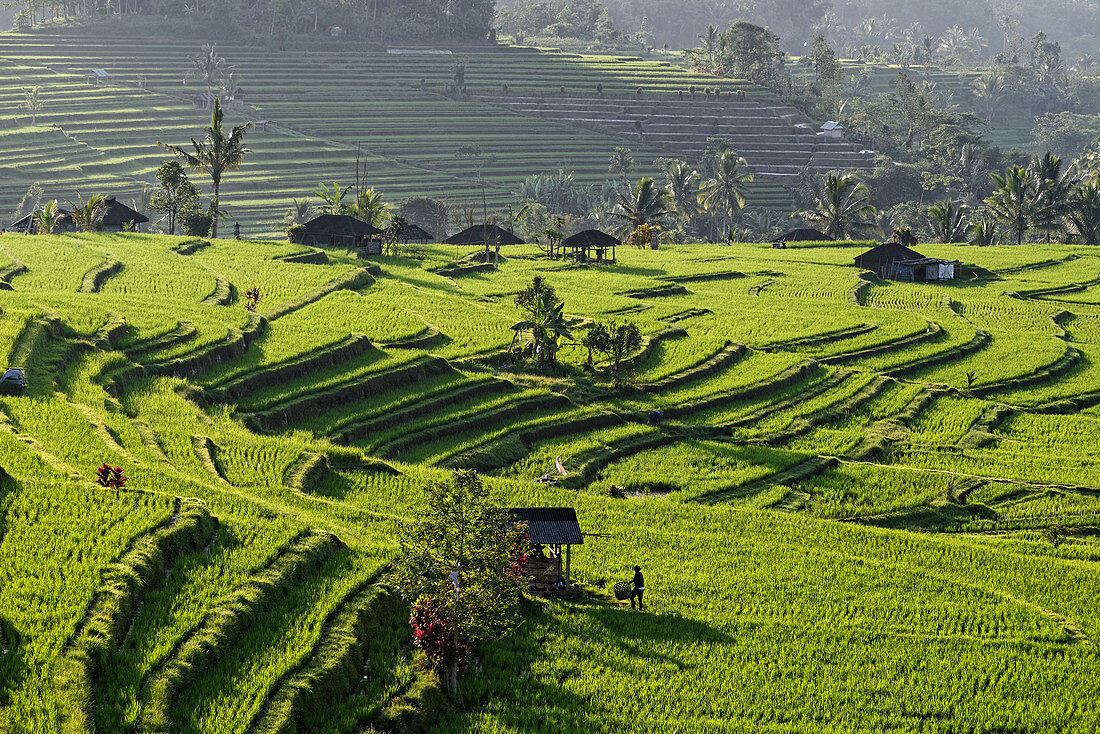This stunning photograph captures the vivid landscape of terraced farmland, possibly located in an Asian country. Dominating the lower two-thirds of the image, the terraces are painted in an intense and lively green, creating a visually striking effect. The terraces, reminiscent of little stair steps descending from left to right, are meticulously manicured and exude a sense of care and maintenance.

Scattered across the farmland, there are various huts and work sheds where workers are seen carrying large baskets, likely filled with harvested produce. In the foreground, a person is visible, carrying what might be a wheelbarrow or another piece of farming equipment, adding a human element to the serene landscape. While the primary focus appears to be on grass or possibly soy, some suggest it might even be a rice paddy.

Background terraces extend into shadow, giving them a slightly darker hue. The scene is dotted with palm trees and an array of flowers, adding bursts of color and life to the predominantly green setting. Natural daylight bathes the entire landscape, highlighting the well-maintained and lush environment. The photograph exudes a sense of calm and showcases the beauty and functionality of terraced farming.